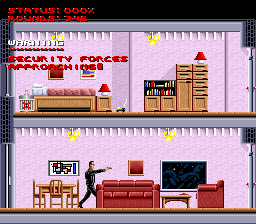This image appears to be a screen capture from a retro-style video game featuring two-dimensional, cartoonish graphics. It showcases an open interior view of a structure, bordered by dark edges. The structure has two levels with distinctive design elements. The walls of both levels are painted in a lavender hue, while the floors and ceilings are demarcated by three gray horizontal lines.

The top level features light brown furniture, creating a contrast with the pinkish walls. In contrast, the bottom level is furnished with reddish-brown pieces. Dominating the lower level is a character, seemingly a white male, dressed in dark clothing. He is holding a gun pointed towards the right side of the image, suggesting he is ready for action or in the midst of gameplay.